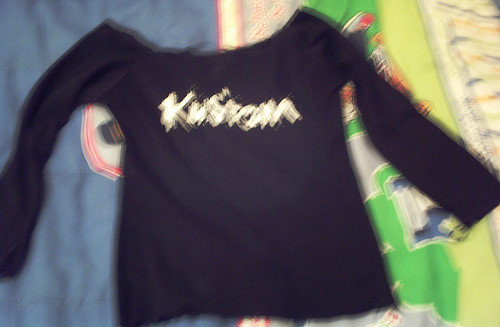This is a very blurry photograph capturing a long-sleeve black shirt hanging in front of a wall adorned with various decorative elements. The shirt prominently features white text, although the blurriness makes it difficult to decipher; it appears to potentially spell out "K-U-S-T-O-N" or something similar. The backdrop includes a visually divided wall, with one side featuring a blue hanging, possibly shaped like a shield, and the other side displaying medium and light green hangings with indistinct designs partially obscured by the shirt’s sleeves. Overall, the image's lack of clarity hampers the ability to discern fine details.